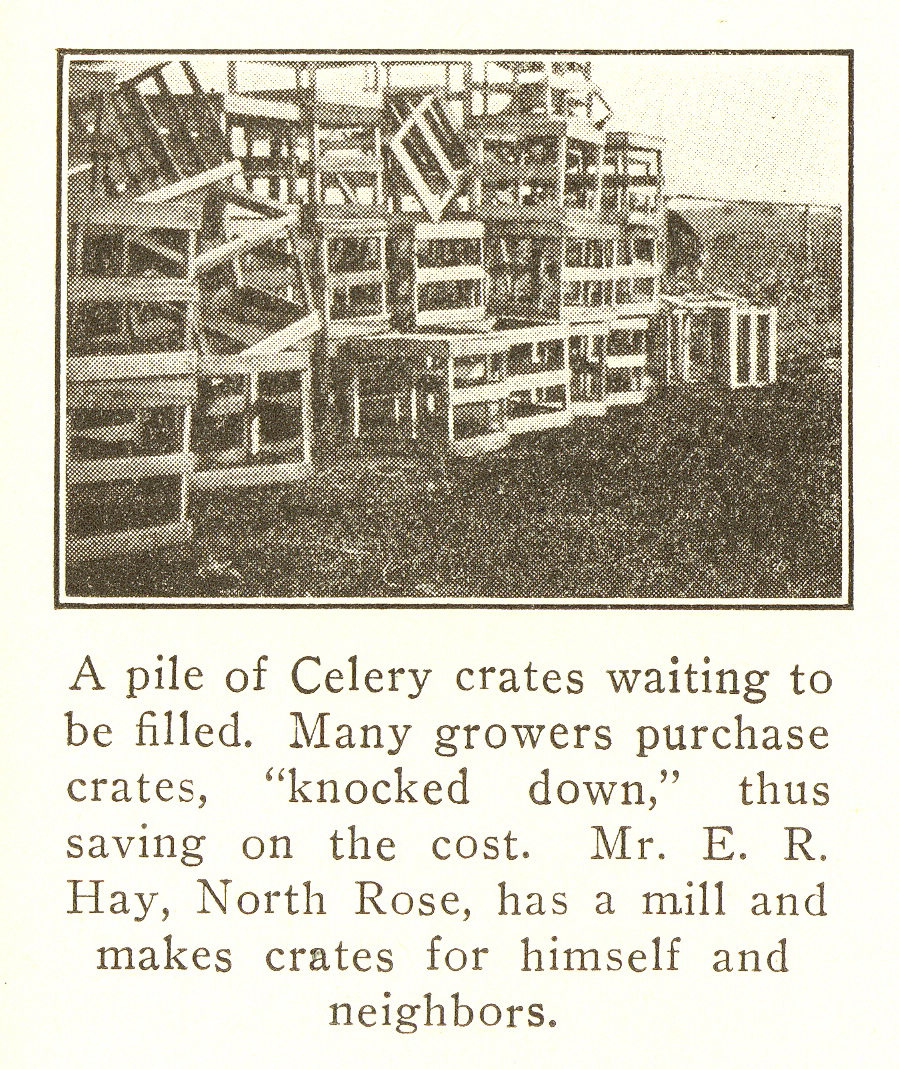This image is an old, grainy black-and-white photograph, reminiscent of a newspaper clipping, showing a cluttered outdoor field filled with empty celery crates. The crates are stacked haphazardly, with some properly aligned and others awkwardly leaning or falling over. The worn-out appearance of the image adds to its rustic quality, capturing a moment in agricultural history. Below the photograph, a caption explains, "A pile of celery crates waiting to be filled. Many growers purchased crates knocked down, thus saving on the cost. Mr. E. R. Hay, Norse Rose, has a mill and makes crates for himself and neighbors." This detail highlights the practical measures farmers took to minimize expenses and the communal support within the farming community.